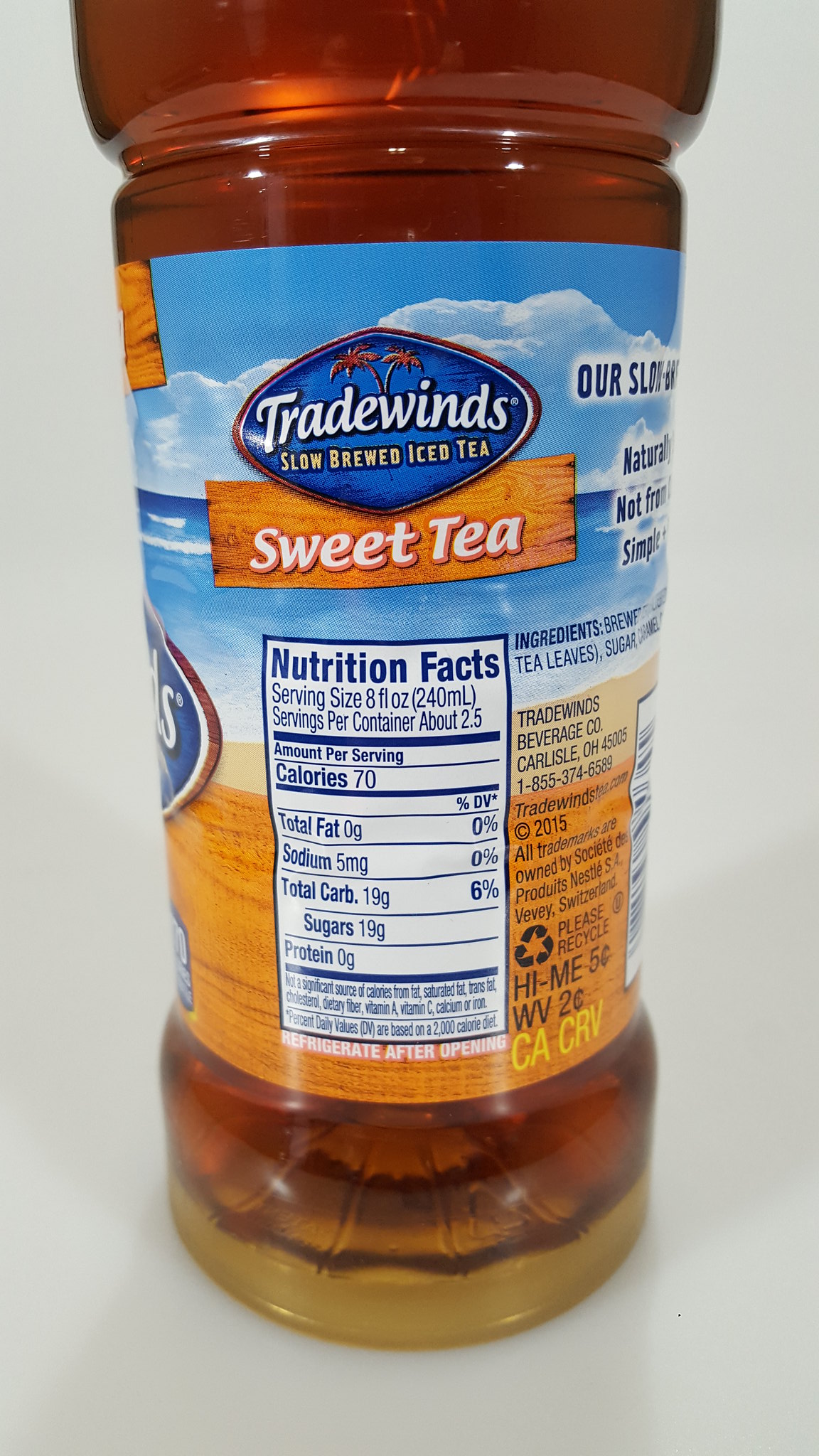This detailed caption describes the Nutrition Facts label on a beach-themed plastic bottle of iced tea.

---

The Nutrition Facts label is prominently displayed on the side of a plastic bottle of iced tea, conveying a beach motif. The label is designed to resemble a quaint piece of driftwood. Above the nutrition information, the label creatively features the product name "Sweet Tea" and the brand "White Fawn" in a visibly relaxing, sun-washed style. Additionally, a distinctive oblong circle at the top of the label reads "Trade Winds Slow Brewed Iced Tea." The fluid inside the bottle is a translucent brownish color with a slight yellow tint, hinting at the refreshing and natural ingredients of the iced tea.